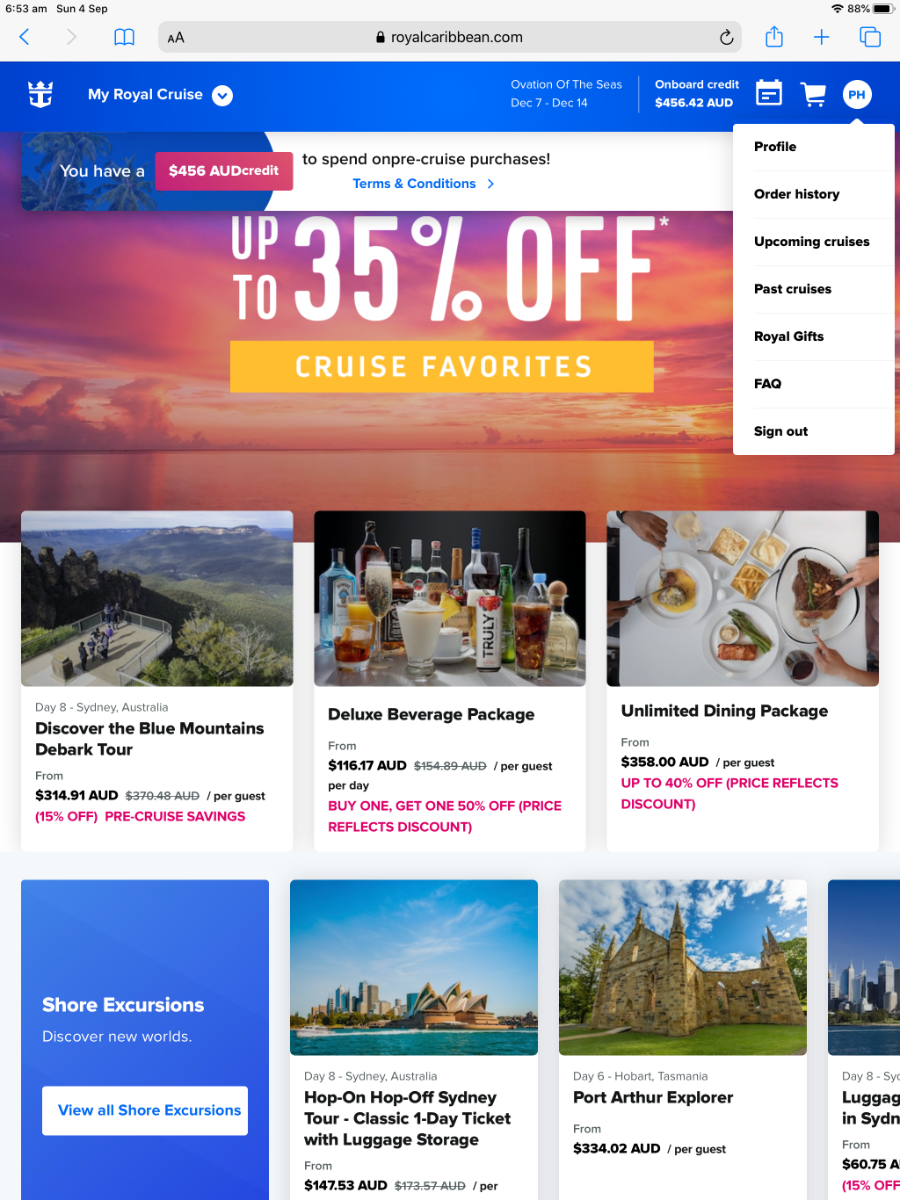In this image, we see a detailed screenshot from a tablet displaying a webpage from RoyalCaribbean.com. In the upper left corner, black text indicates the time as 6:53 a.m. on Sunday, 4th of September. The upper right corner shows the Wi-Fi icon and a battery icon indicating an 88% charge.

Below, there is an address bar showing RoyalCaribbean.com. Directly beneath the address bar is a blue banner featuring the Royal Caribbean logo, a white crown, and the text "My Royal Cruise" with a pull-down arrow. To the right, it lists "Ovation of the Seas" with the dates "December 7th through December 14th" and onboard credit amounting to $456.42 AUD. Additionally, the banner includes an icon for a shopping cart and a circular icon with the letters "PH" indicating a profile. The pull-down menu beneath the "PH" icon displays several options: Profile, Order History, Upcoming Cruises, Past Cruises, Royal Gifts, FAQ, and Sign Out.

The background of the screenshot features a stunning sunset over the water, adding a serene and picturesque backdrop to the overlaying elements. Across this sunset scene, in bold white text, it reads "Up to 35% Off Cruise Favorites," highlighting a promotional offer.